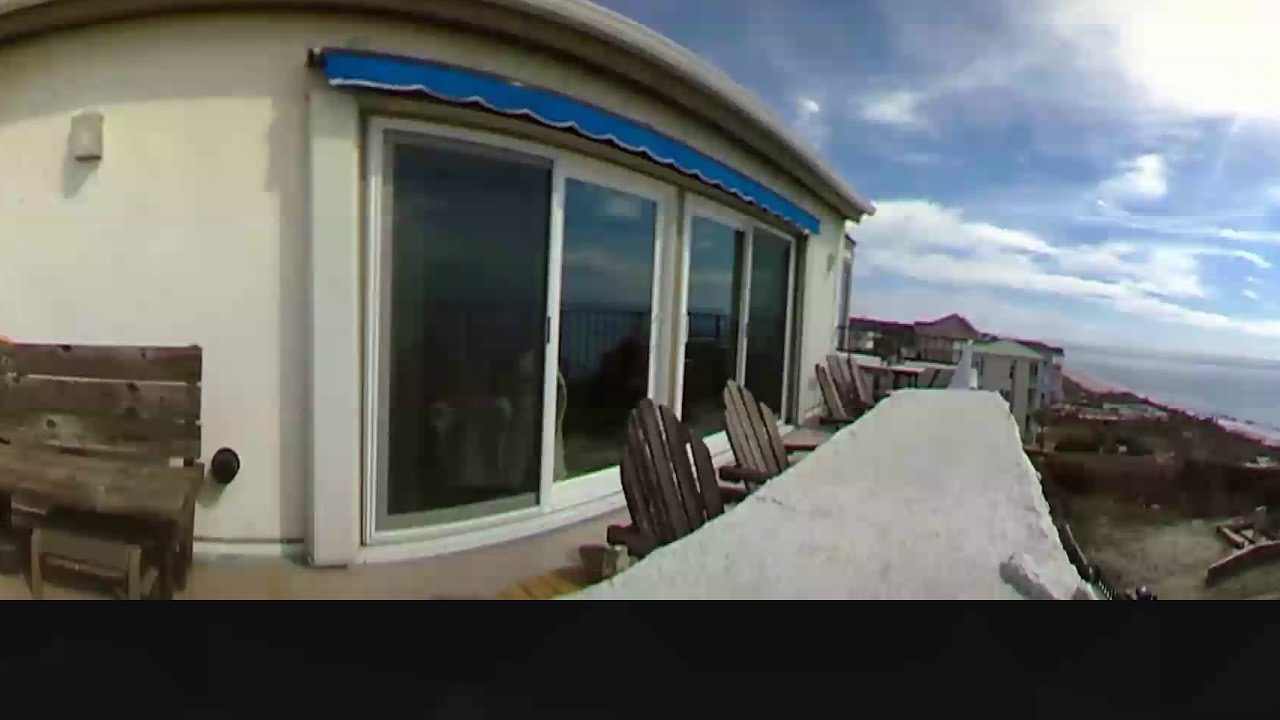The image captures the sunny daytime view of a raised patio area on the upper level of a white beachside residence, likely located along the Mediterranean coast. The patio features three wooden slatted chairs positioned in front of a wide white wall with two vertically-structured sliding glass doors, framed in white, and adorned with a royal blue canopy. On the left side, leaning against the light beige exterior wall, is a wooden bench. The patio has a concrete or alabaster fence which overlooks neighboring buildings—a series of white and red residences—and stretches to reveal a glimpse of the ocean on the far right. The sky above is a bright blue, dotted with a few wisps of clouds and illuminated by the sun in the upper right corner, creating a slight glare.